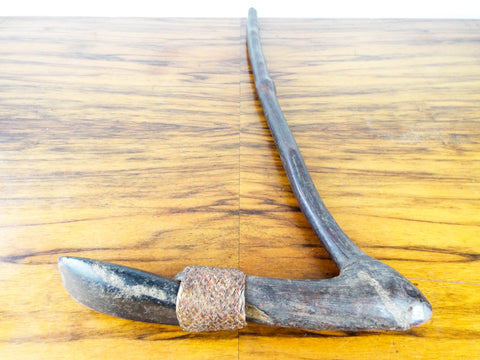The photograph is a smaller, horizontally-aligned rectangle with no border or text, depicting a metal tool that resembles an archaic wishbone or a large clamp. This v-shaped object, with metallic shades of silver, gray, black, white, and brown, lies on a medium to dark brown wooden surface featuring prominent horizontal wood grains. The tool appears professionally photographed under good lighting, though its exact nature remains ambiguous—whether it's naturally occurring or crafted in a metal shop is uncertain. The tool consists of two pieces, with the left part being wider and horizontal, while the right part is thinner and reaches a point before extending straight leftwards. A golden or grayish-brown band, possibly akin to a band-aid, wraps around the intersection where the two pieces meet.